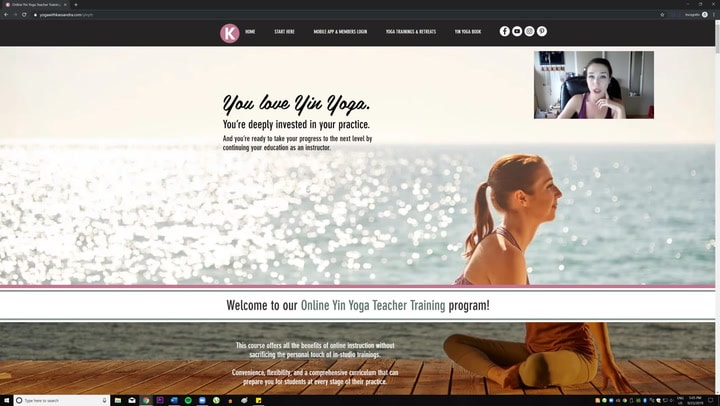This screenshot is taken from a website showcasing a live stream meeting. In the top-right corner, there is a small rectangular video window displaying a woman seated at a desk, engaged in conversation with the camera. She is clad in a purple yoga tank top. The website prominently features an image of either the same woman or someone resembling her, with brown hair secured in a ponytail, executing a yoga pose. The background of this image reveals the glimmering lights of a vast ocean. Overlaying the horizon in black text, the message reads: "You love yin yoga. You're deeply invested in your practice." Subtext further elaborates: "You're ready to take your progress to the next level by continuing your education as an instructor." At the bottom of the page, a banner announces: "Welcome to our online Yin Yoga Teacher Training Program." This indicates that the website offers a course for individuals aspiring to become certified yin yoga instructors.